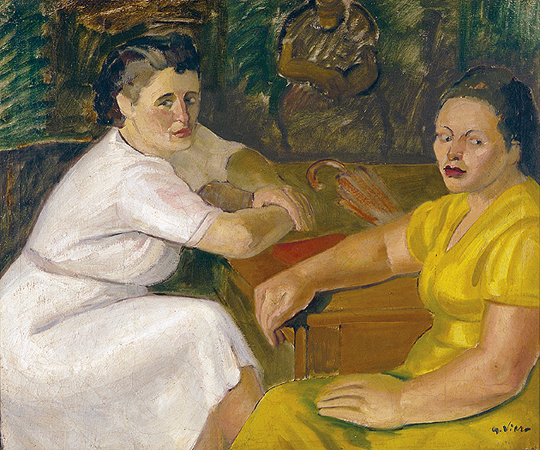The image portrays a detailed and colorful painting featuring two women sitting at a table. Both women have dark hair and are adorned with red lipstick. The woman on the left is dressed in white and has both her arms resting on the table, while the woman on the right is in a yellow dress with one arm on the table and the other in her lap. The table is adorned with a red book and an orange and white umbrella. The background is less detailed and features a murky palette with sharp, directional strokes in green and yellow, creating a contrasting texture to the more defined foreground. Slightly obscured in the background is another woman sitting on a chair, though her head isn't visible. The women in the forefront appear to have been interrupted, with one looking cautiously off to the side and the other gazing outward, giving an air of worry and intense contemplation. Their expressions, combined with the rapid and less detailed brush strokes of the background, suggest a scene of tension or anticipation, as if waiting for something momentous to occur.